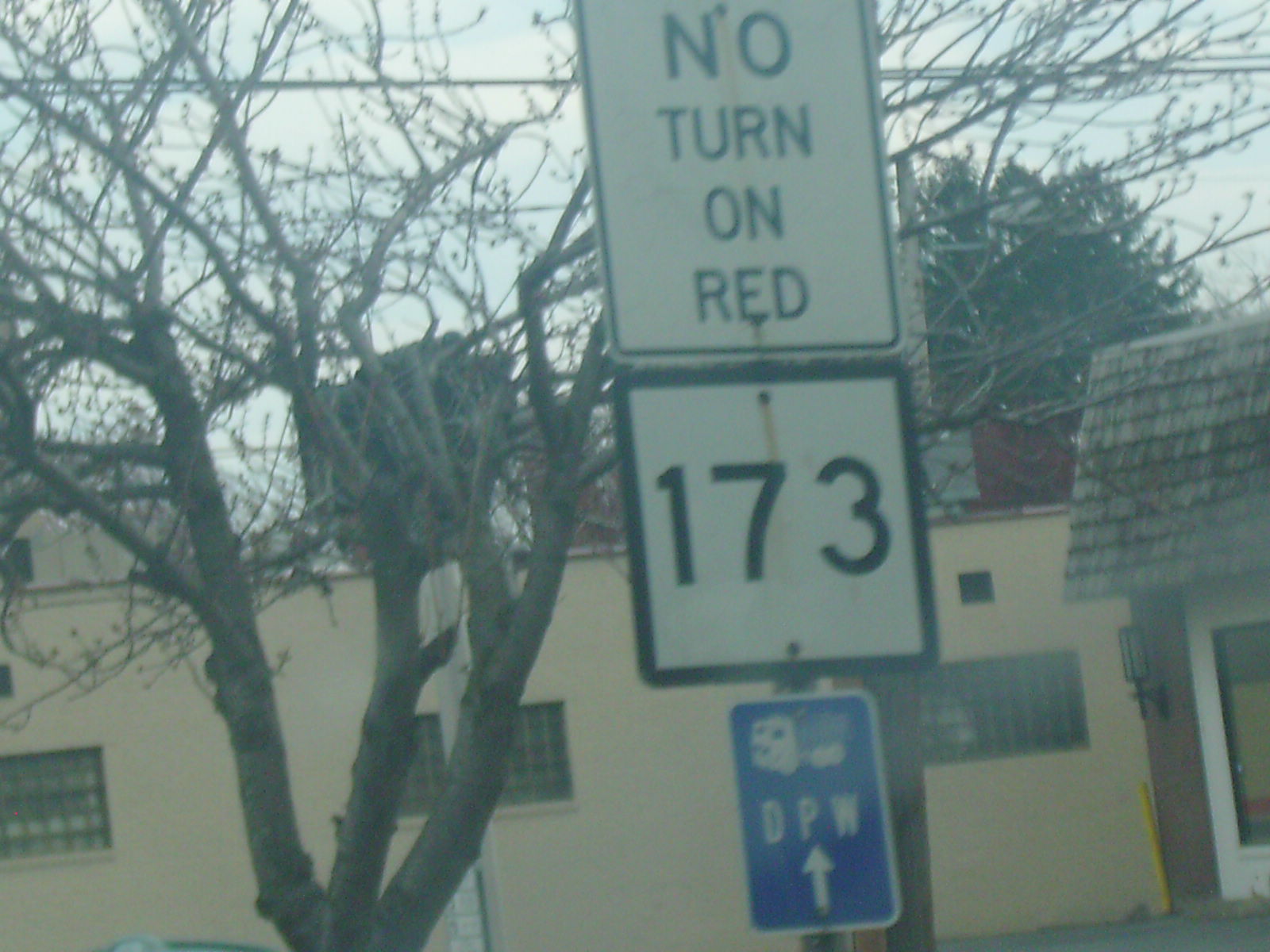A color photograph captured outdoors on a slightly hazy day features a central white road sign edged with a thin black border. The sign prominently displays "NO TURN ON RED" in capital black letters. Directly beneath it, a red square sign with a thicker black border shows the number "173." Below the red sign, a rectangular, blue sign oriented lengthwise includes the acronym "DPW" and an upward-pointing arrow. To the left of the signs, a red brick building with a cedar-shaped roof is visible, partially obscuring a tan, elongated building in the background. The sky above is a clear blue, and the foreground is dotted with numerous leafless trees, adding a bare, wintry feel to the scene.